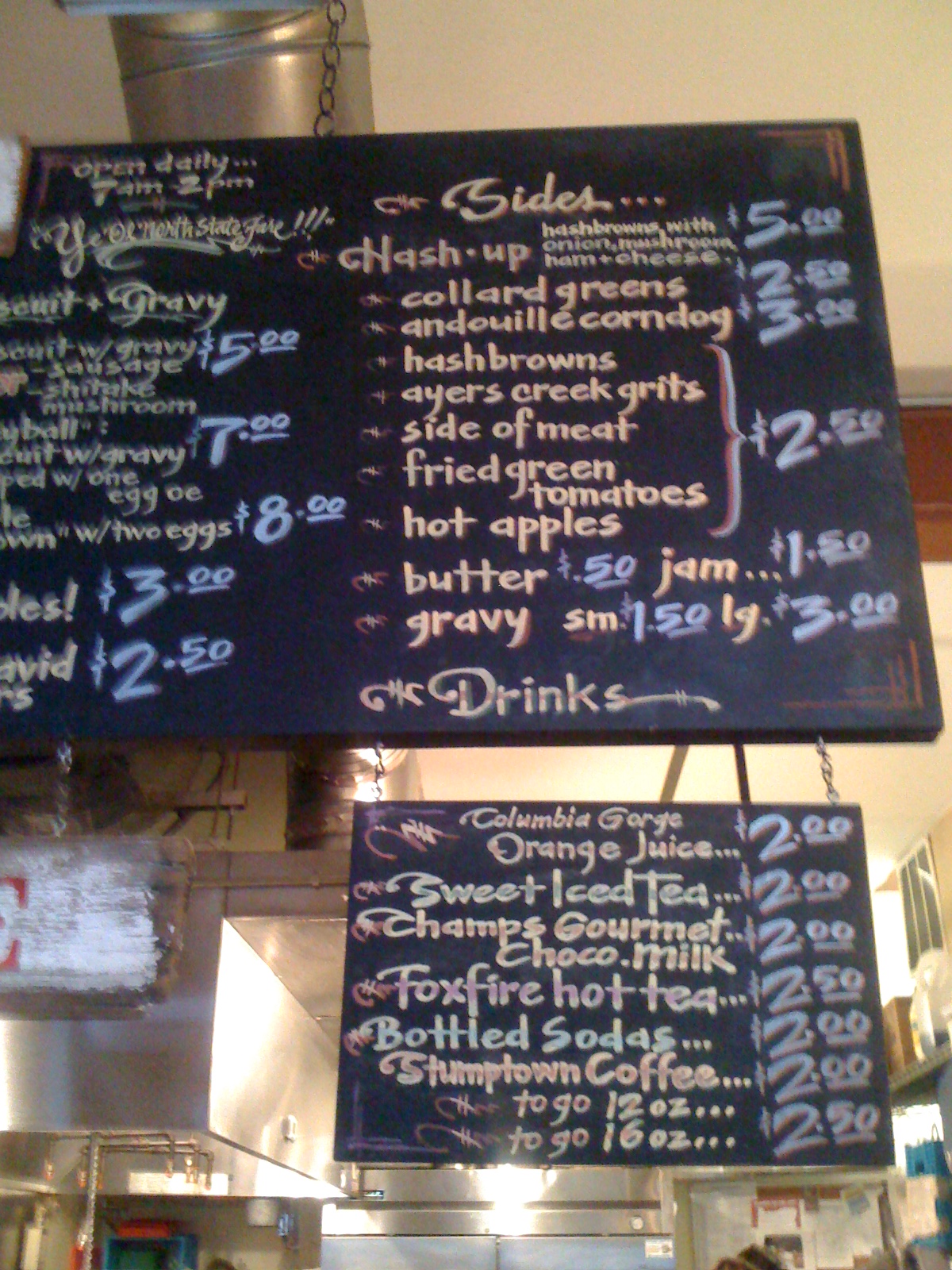A detailed view of a restaurant's menu board hanging prominently over the counter captures the charm of the establishment. The background reveals an industrial kitchen, characterized by a very high ceiling adorned with lighting, ample storage, and exposed pipes, though the actual counter remains just outside the frame.

The main menu is sizable and designed in a classic black chalkboard style, divided into two columns of offerings. The left column is headlined with "Open Daily, 7 a.m. to 2 p.m." and "Ye Olde North State Fare." This section lists a variety of hearty dishes, including biscuits and gravy, meatball with biscuit and gravy, a partly visible two-egg dish, and two other items that are cut off. The menu items are written in a beige-brown hue, accompanied by prices: $5, $7, $8, $3, and $2.50.

The right column is dedicated to sides, featuring an enticing assortment: hash-ups, collard greens, andouille corn dog, hash browns, Ayer's Creek grits, side of meat, fried green tomatoes, hot apples, butter, jam, and gravy.

Underneath the larger menu board hangs a smaller sign, tethered by chains, listing the available drinks. The beverages include Columbia orange juice, sweet iced tea, Champ's gourmet chocolate milk, Foxfire hot tea, bottled sodas, and Stumptown coffee, with pricing consistently set at either $2 or $2.50. The detailed arrangement of menu items and prices offers a comprehensive glimpse into the culinary delights awaiting patrons.